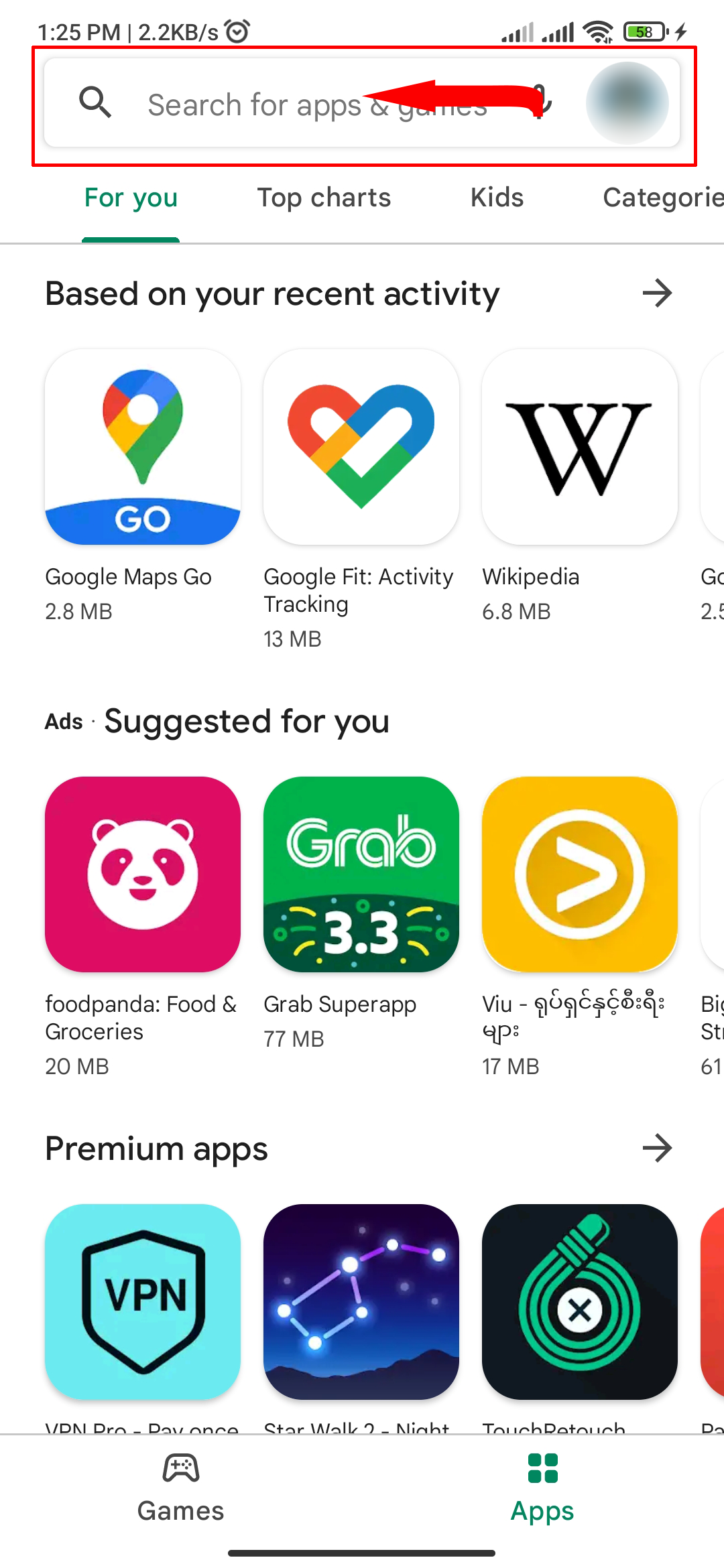A detailed screenshot of a cell phone app store interface:

The background of the app store is predominantly white. At the very top, there is an extensive search bar stretching across the entire width of the screen. Inside the search bar, the text "Search for apps & games" appears in small gray letters, accompanied by a magnifying glass icon on the left. To the far right, there is a circular user profile icon that is currently grayed out.

Underneath the search bar, there is a vertical list of categories, which includes options like "For you," "Top charts," "Kids," and "Categories." The "For you" category is selected, indicated by blue highlighted text and a matching horizontal blue line beneath it. At the top of this section, bold black text reads "Based on your recent activity," accompanied by a right-pointing arrow.

Below this, a horizontal row of app icons is displayed:
1. The first app is "Google Maps Go," with its size listed at the bottom left below the title.
2. The second app is "Google Fit: Activity Tracking," also with its size noted in the same position.
3. The third app is "Wikipedia," followed by an arrow pointing to the right above the icon, suggesting the category can be expanded to view more apps.

Further down, the text "Ads" appears in small black font on the left, next to "Suggested for you," with once again, a horizontal listing of app icons displayed.

Continuing downward, the bold black text "Premium apps" is positioned at the top left, followed by another horizontal arrangement of app icons.